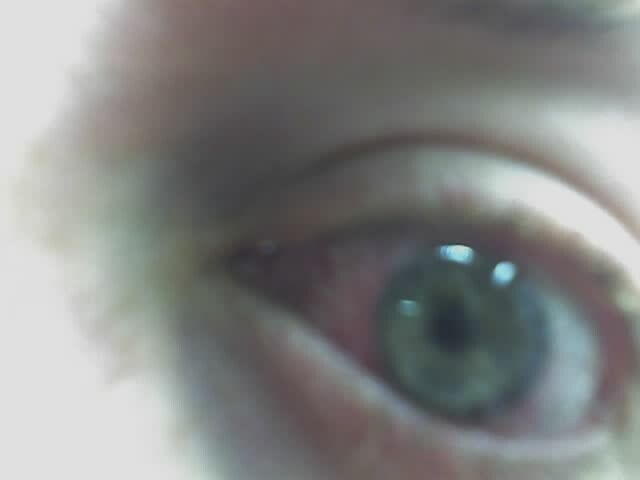This is an extreme close-up image of a human eye, primarily focused on the iris and surrounding areas. The eye is predominantly green, with a gradient that transitions to a bluish green towards the outer edge of the iris. The inner part of the iris closer to the pupil shows a more vivid green hue. The image is notably blurry and overexposed, possibly due to a harsh flash that casts a glaring white light on the bridge of the nose and parts of the eyelid. This intense lighting makes finer details difficult to discern. The eye appears slightly bloodshot, with visible red veins, particularly on the left side near the tear duct. Bits of the eyebrow and eyelashes are visible, and there's no sign of makeup. The person seems to be Caucasian, and the wide-open eye reflects some white spots from the flash.